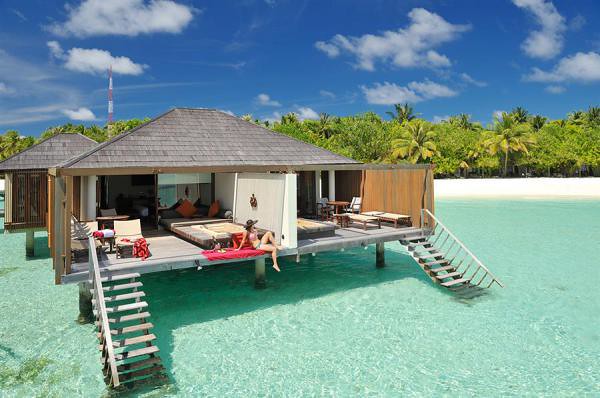This photograph captures a picturesque tropical beach resort scene with incredible detail. Dominating the image are luxurious beach cabanas perched on stilts over crystal-clear, sea-green water, creating an idyllic and serene setting. Each duplex cabana features spacious wooden decks with large glass windows that offer stunning views of the surrounding beach and ocean. White stairs descend from the decks directly into the shimmering water. 

Central to the image is a woman in a bikini, lounging on a red blanket on the deck of one of the cabanas, enjoying the sun and the peaceful surroundings. The beach in the foreground is a pristine stretch of white sand, extending toward the right-hand side of the image where it meets a line of lush, light green palm trees and other tropical foliage, creating a natural, jungle-like backdrop.

Above, the sky is a brilliant blue adorned with fluffy, white clouds, adding to the overall charm and tranquility of the scene. In the distance, partially obscured by the palm trees, a radio or cell tower pokes through the greenery, hinting at a blend of natural beauty and modern convenience. The cabanas have triangular gray roofs and are designed with open, airy rooms that merge seamlessly with the outdoor environment, providing a secluded, peaceful escape for guests. This photograph beautifully encapsulates the luxurious and serene essence of a tropical beach villa.